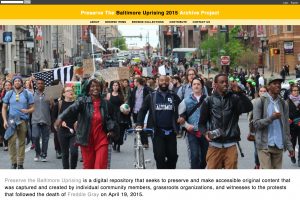A vibrant street scene unfolds before the viewer, with hundreds of people bustling about, signifying the collective energy of a large crowd. This image captures a significant event: the preview of the "Singapore Uprising 2015 Articulate Project." The top of the image is framed with a striking yellow border that draws attention and is complemented by bold white and black text, repeating the event's title. This repetition in the border emphasizes the importance and excitement surrounding this notable cultural initiative.